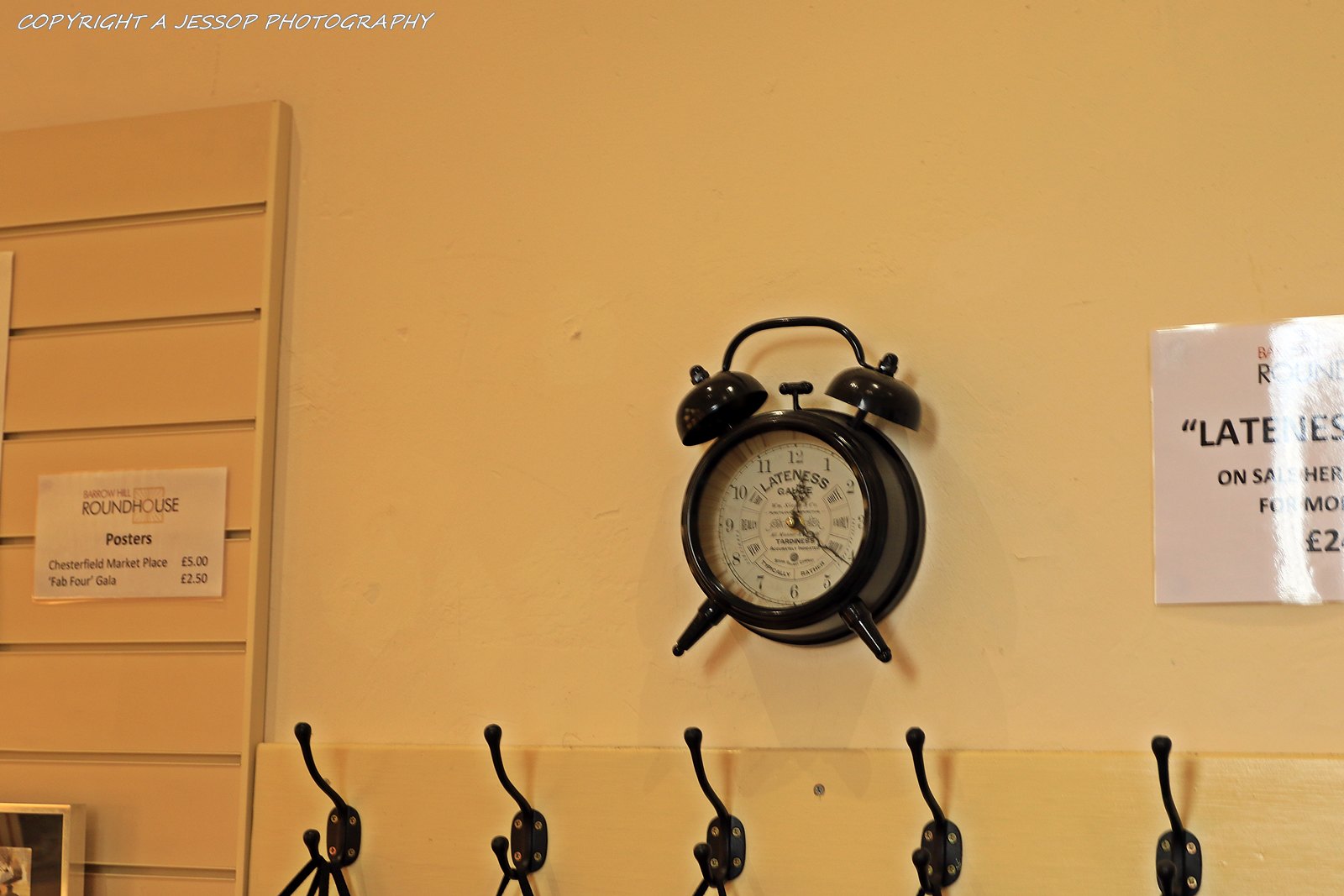This color photograph captures a vintage-style, antique wall clock prominently mounted on an orange wall. The clock, reminiscent of old alarm clocks, features a white face with black numerals and hands, encased in a round black metal frame. It is distinguished by its two dome-shaped black alarms on either side at the top, connected to a handle. Below the clock, there is a row of black hooks, some of which have black cords hanging from them. To the left of the clock and hooks, there is a panelled board displaying a white sign with text that is too small to read and an edge of what appears to be another photograph or picture, framed in black. Additionally, a partially visible sign on the right side is illuminated, making the letters "L-A-T-E" and some black writing, possibly including pound signs, legible. At the upper left corner of the image, white text reads "copyright a Jessop photography."